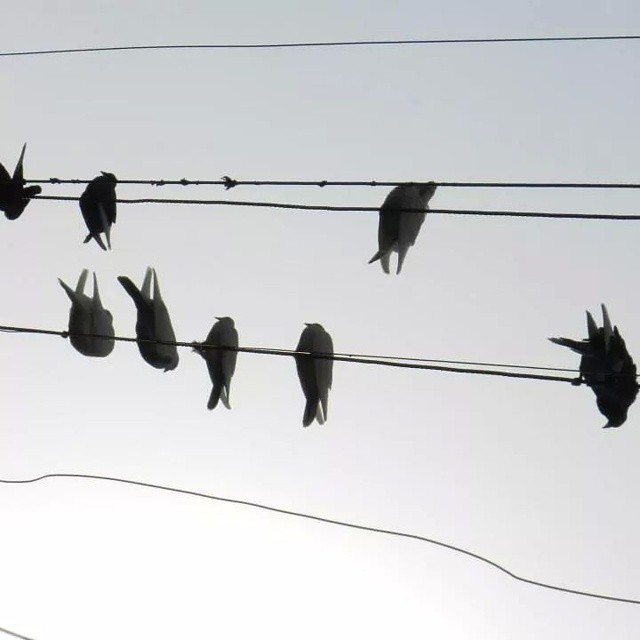This photograph captures a striking image of several silhouetted birds perched on telephone wires against an overcast, gray sky. From top to bottom, the image features a series of six electrical wires. The topmost wire is thin and perfectly straight, while the wire beneath it is thicker and appears slightly frayed, possibly from the birds pecking at it. On this thicker wire, three birds are positioned: two towards the left and one just right of center. The next wire below is equally thick but without any fraying, hosting four birds clustered together from center to the left and one solitary bird on the far right. Beneath them, another thin wire is notably bent on both ends. An additional small piece of wire is visible in the very bottom left corner. The birds, likely crows or dark-colored species, are silhouetted, preventing clear visibility of their colors, with some sitting in standard positions while a few appear to hang in unusual orientations. The overall ambiance is further accentuated by the misty, gradient sky, fading from a darker gray at the top to a lighter hue near the bottom.